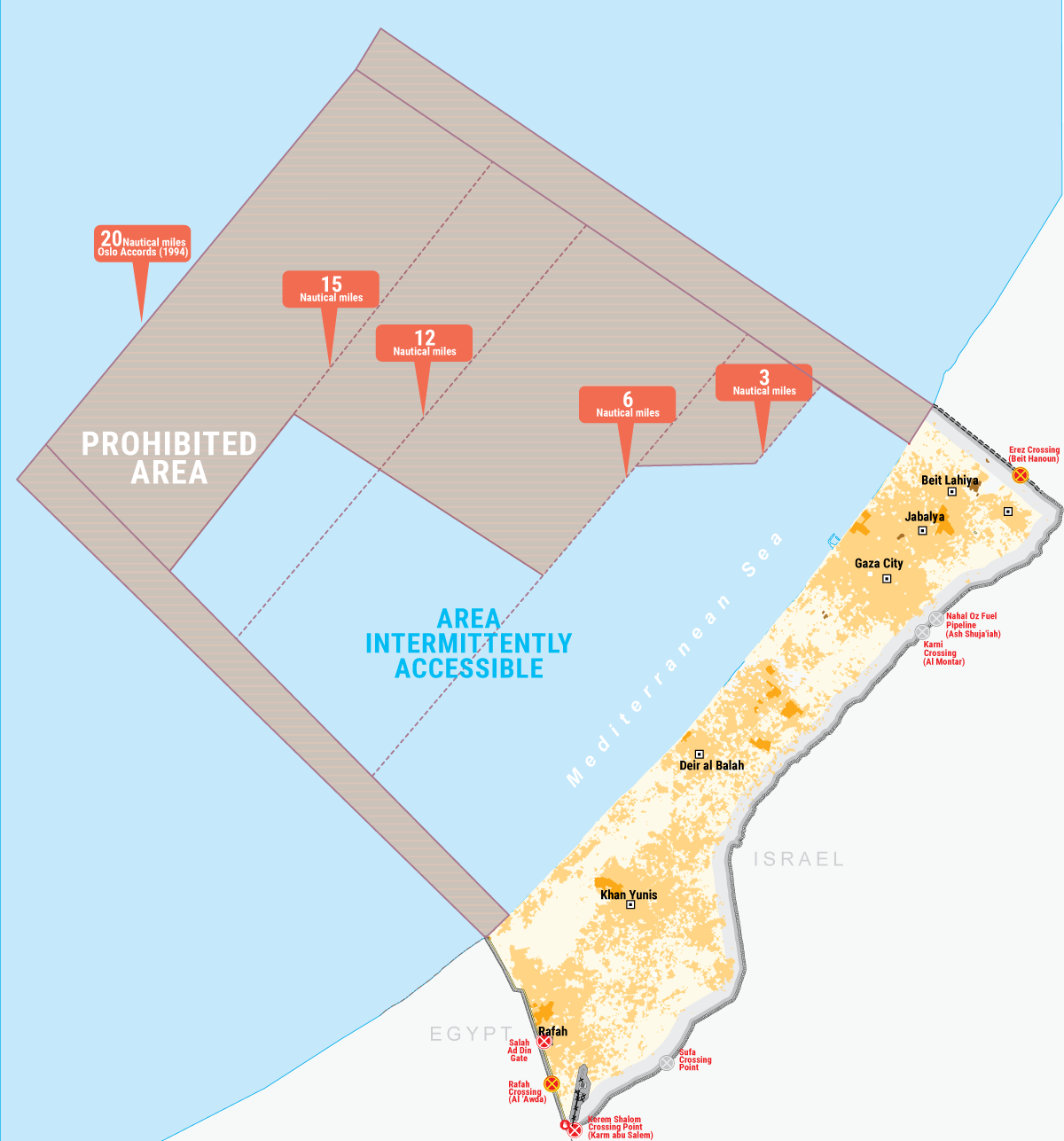The image features a detailed map of a segment of the Mediterranean coastline adjacent to Israel and the Gaza Strip, highlighting various nautical restrictions. The Mediterranean Sea is situated on the left, with the territorial demarcations of Egypt and Israel, including notable locations like Gaza City, displayed on the right. The map prominently marks several areas with prohibitive and restrictive overlays: a gray-shaded area indicates a prohibited zone extending up to 20 nautical miles offshore, segmented by lines at 15, 12, 6, and 3 nautical miles. Within these segments, the area between 3 to 12 nautical miles is intermittently accessible, illustrated in a distinct pattern. Additionally, various texts in black denote city names, while red text provides critical notations around the map's border. Noteworthy visual markers include yellow and red colored X icons, one located in the top right and three at the bottom, differing from other map icons.